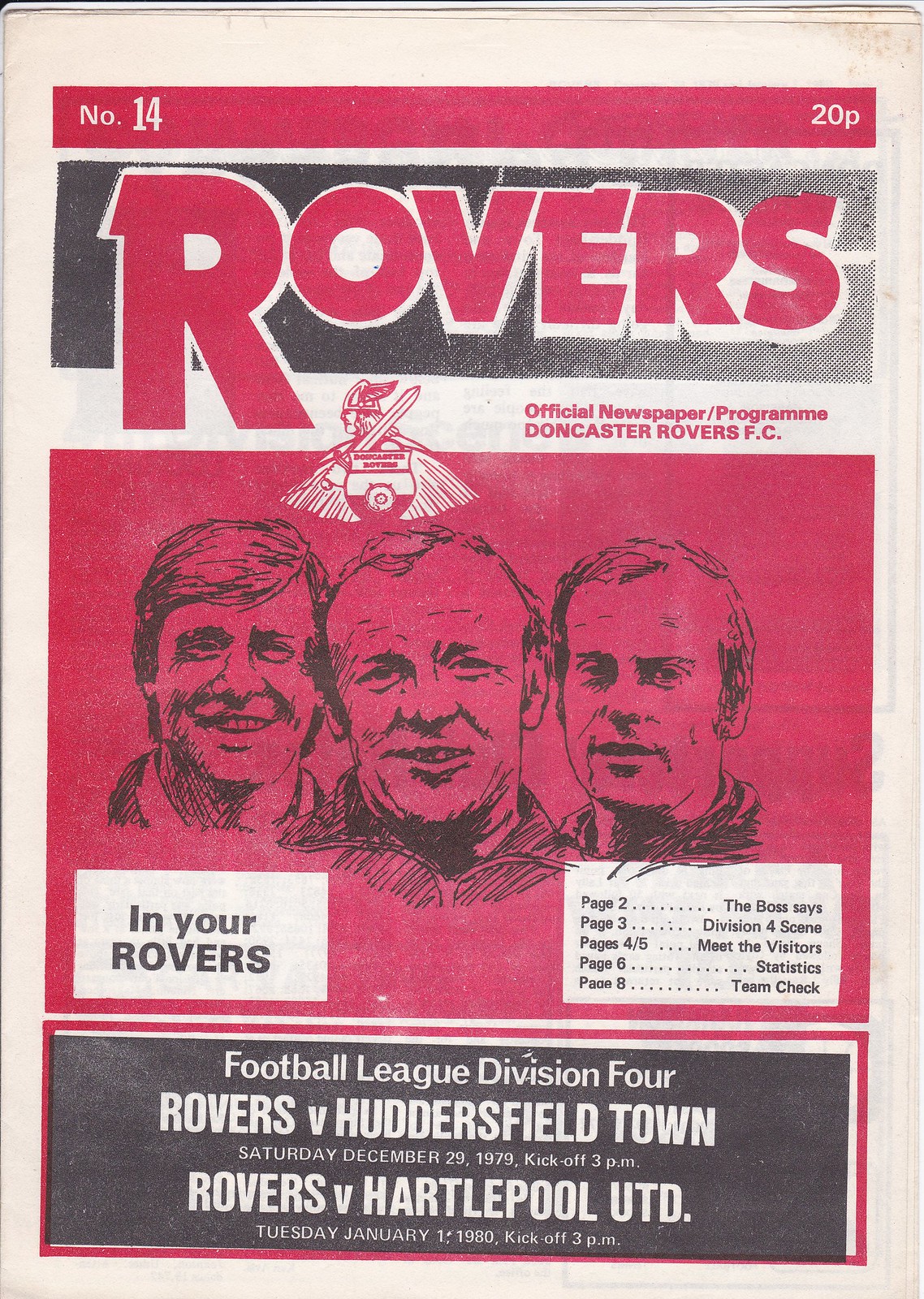The image depicts the front page of a match day program for the Doncaster Rovers FC. The program is on off-white, slightly worn paper, with visible edges at the top and additional pieces layered behind. At the very top, a red rectangle stretches across, displaying "No. 14" on the left in bold white letters, and "20P" on the right.

Below this, a black rectangle fades into grey on the right, featuring a prominent red text that reads "ROVERS," outlined in white. Directly beneath this is another large red rectangle that dominates the center of the page. It includes black line drawings of three smiling men, likely players, sketched in pencil. The drawings are set against the red background and appear in the center, with one man in the middle and two on either side.

To the left of these sketches is a small white rectangle stating "In your Rovers" in black letters, while another white box to the right details page listings from the program, such as:
- Page 2: The Boss Says
- Page 3: Division Four Seen
- Pages 4/5: Meet the Visitors
- Page 6: Statistics
- Page 8: Team Check

At the bottom of the front page, a black rectangle contains white text noting the match details:
"Football League Division Four
Rovers vs. Huddersfield Town
Saturday, December 29, 1979, Kickoff 3 p.m. 
Rovers vs. Hartlepool United 
Tuesday, January 1980, Kickoff 3 p.m."

The program signifies an official event publication from the Doncaster Rovers FC, complete with their Viking logo featuring a Viking with a sword on his shoulder, looking to the left.